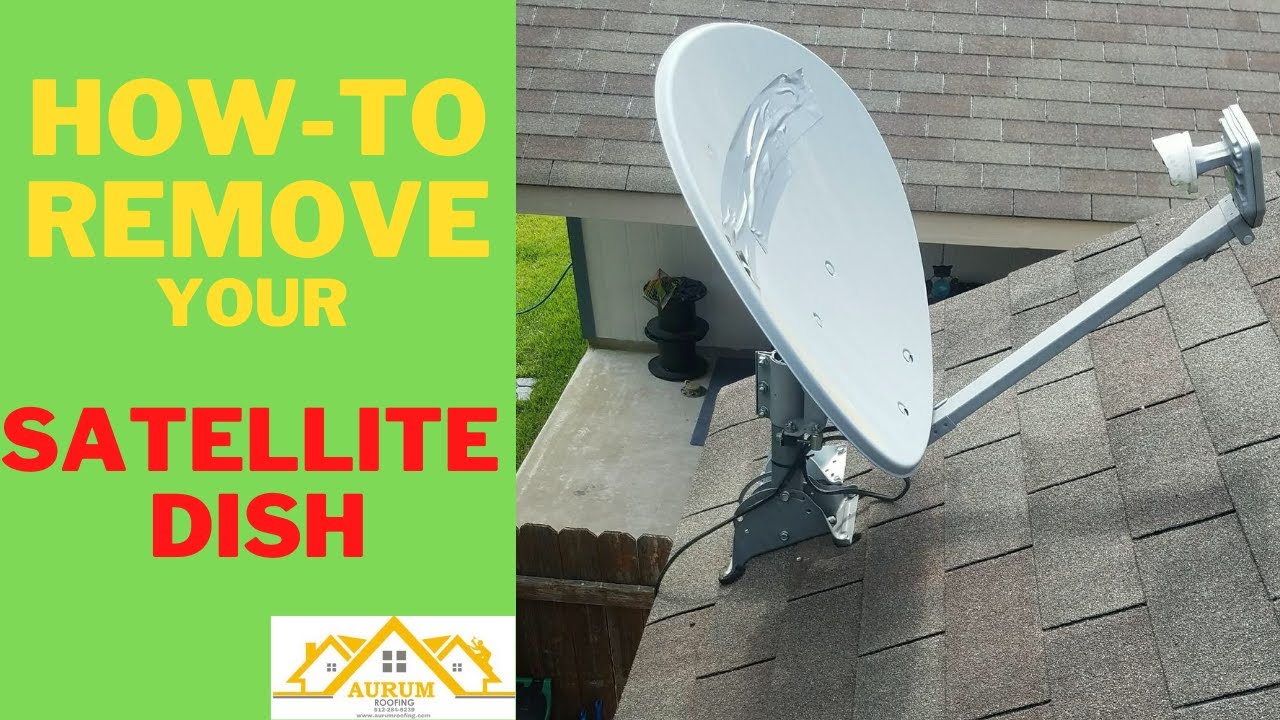The image is a detailed, brochure-like guide on how to remove a satellite dish. The left third of the image features a solid lime green background with bold text in yellow and red reading, "How to Remove Your Satellite Dish." The bottom corner of this section displays the Aurum Roofing logo, depicting a group of yellow houses, accompanied by a phone number and website in small text. To the right, the remaining two-thirds of the image illustrate a white satellite dish mounted on a new-looking, gray-tiled roof. The dish, which faces to the right, is secured with bolts and has wires trailing off below the roof. Notably, there is some duct tape on the dish. In the background, there is a view over the fence to another house without a satellite dish. Bright green grass is visible along the bottom of the image, contributing to the fresh, clean visual layout.